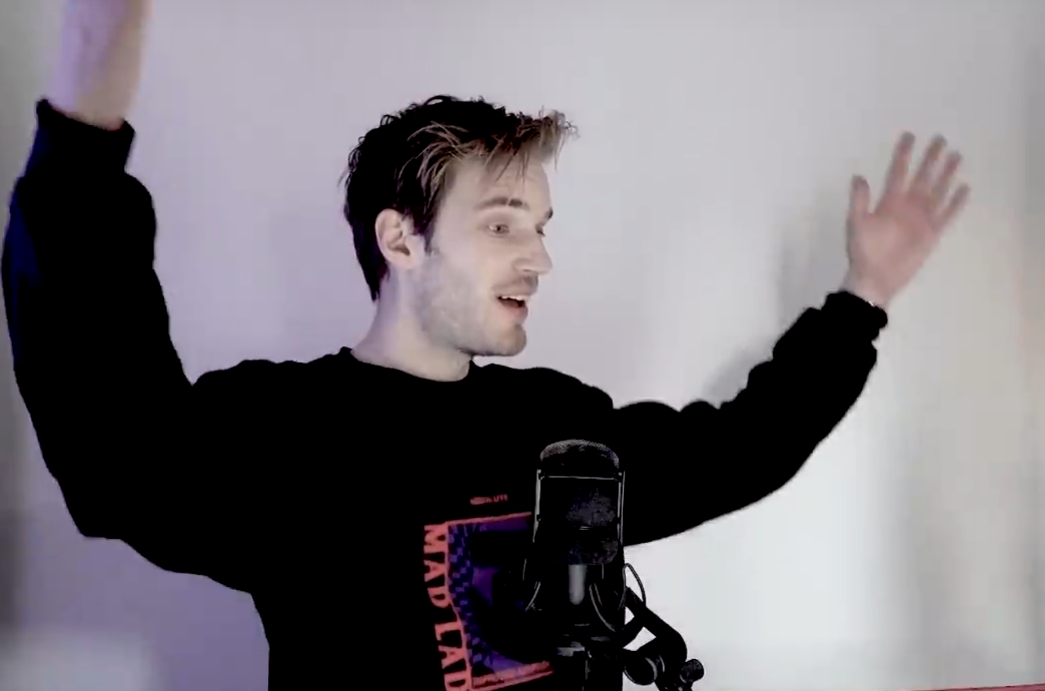In this slightly blurry screenshot from a YouTube video, the famous YouTuber PewDiePie is captured. He is dressed in a black sweatshirt with the yellow phrase "Mad Lad" prominently displayed on the chest. PewDiePie's black hair is stylishly accentuated with frosted tips, and he has a bit of five o'clock shadow on his face. His expressive blue eyes are directed to the right, offering a glimpse of his right profile. He is sitting in front of a white backdrop, which is faintly shadowed, adding depth to the scene. PewDiePie's hands are raised mid-gesture, appearing blurred due to movement. A large, black, mounted microphone is positioned in front of his sweatshirt. Notably, he displays a set of very white teeth. In the very lower right corner of the image, a slight touch of brown can be seen.